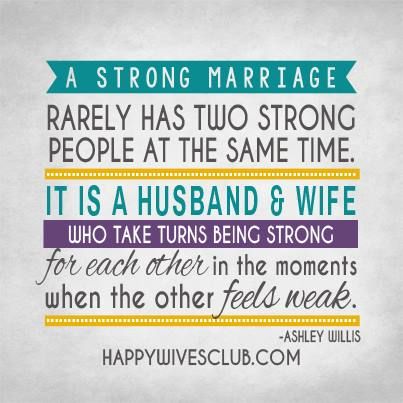The image displays an inspirational sign with a gray and white background from happywivesclub.com. At the top, there's a teal rectangle containing the phrase "A strong marriage" in white letters. Following this, in black text, it states, "rarely has two strong people at the same time." 

Proceeding horizontally across the sign is a yellow line adorned with white dots. Below this, in teal letters, it reads, "It is a husband and wife." Directly below this text is a purple rectangle featuring the white-lettered phrase, "who take turns being strong."

Continuing, in black cursive, the words "for each other" are written, followed by "in the moments" in standard black font. Another line of text underneath states, "when the other feels weak," where "feels weak" is also written in black cursive.

Below this statement is another yellow rectangle with white dots running horizontally. At the bottom right corner, "Ashley Willis" is written in black letters, while the center bottom of the sign features "happywivesclub.com" also in black letters.